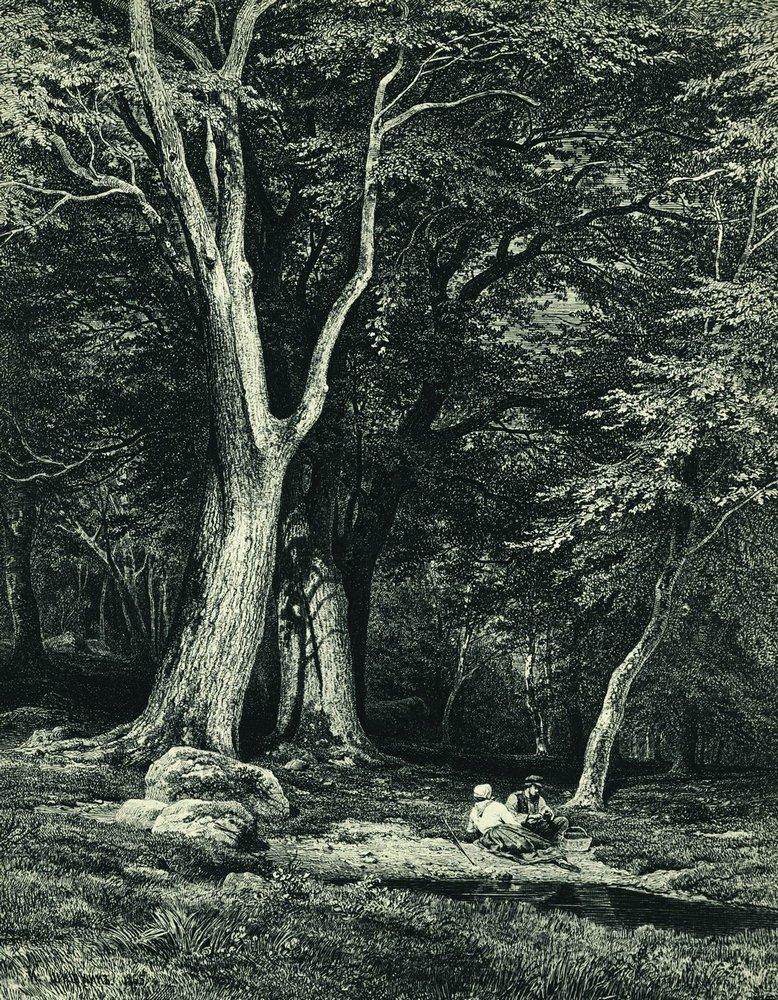In this dark and intricate black-and-white painting, possibly done with pencil or charcoal, the focal scene depicts a dense forest with a subtle, greenish hue. The setting is dominated by two massive, leafy trees situated on the left side, standing majestically before a few large boulders. The forest canopy is thick and full, obscuring the sky and sun, and casts numerous shadows, suggesting a daytime scene. 

In the lower right of the painting, a man and a woman are having a picnic on a grassy patch. The man, wearing a hat, vest, and button-down shirt, is seated with a picnic basket at his feet. The woman, dressed in a long-sleeve shirt and a skirt, reclines on the ground beside him, facing him as though engaged in a quiet conversation. The pair is near a small body of water—possibly a pond, lake, or stream—that reflects the trees. The entire scene is enveloped in the tranquility of nature, with additional trees populating the background and right side, further enhancing the secluded, serene atmosphere.